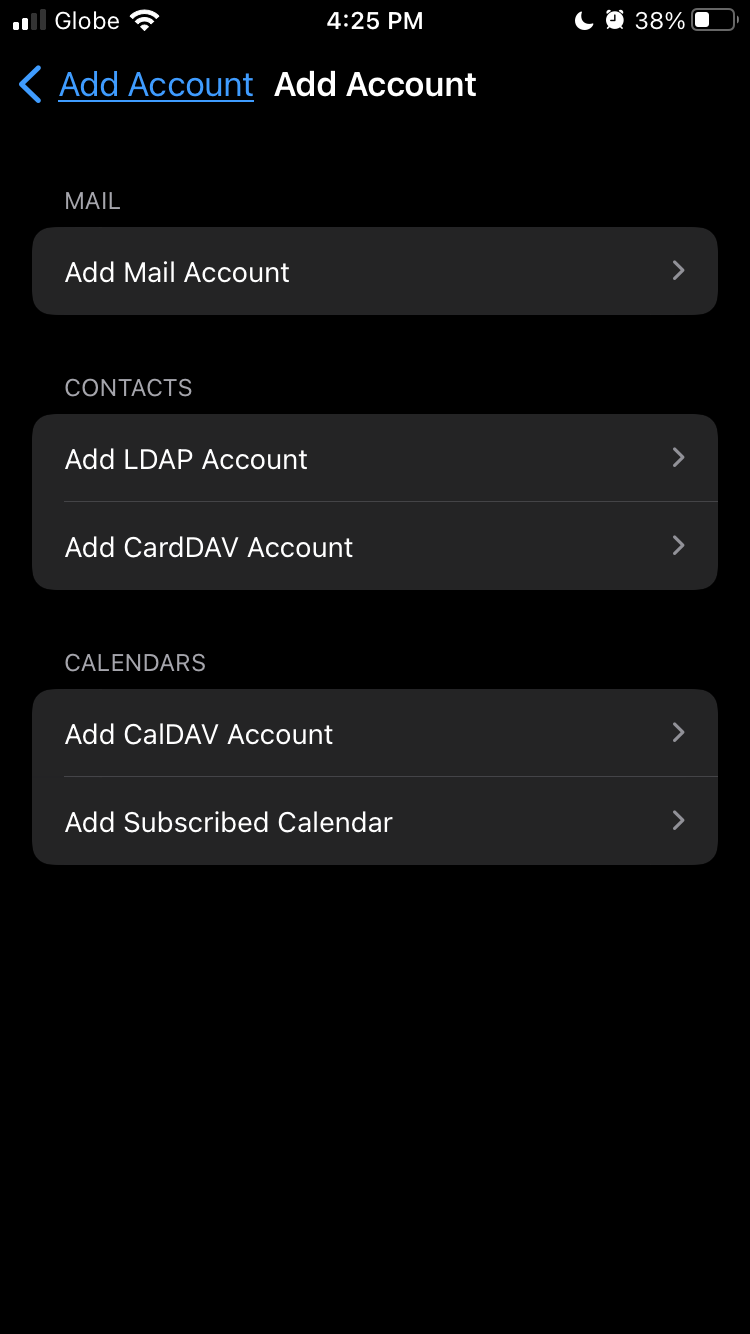This screenshot from a smartphone, featuring a black background, displays several elements of the phone's status and settings. At the top, the status bar indicates two out of four signal bars with "Globe" as the carrier, a Wi-Fi signal icon, the time "4:25 p.m.", an alarm clock icon, and a battery level at 38%.

Below the status bar, there's an interface for adding accounts. At the top of this section, there's a blue "<" symbol followed by the text "Add Account" in white. The options for adding different types of accounts are listed as follows:

1. **Mail**
   - Grey text: "Mail"
   - Below it, a grey box with white text: "Add Mail Account" followed by a ">" symbol on the right.

2. **Contact**
   - Grey text: "Contact"
   - Below it, a grey box with white text: "Add LDAP Account" followed by a ">" symbol on the right.

3. **Add CardDAV Account**
   - Grey text: "Add CardDAV Account"
   - Below it, a grey box with white text: ">" symbol on the right.

4. **Calendar**
   - Grey text: "Calendar"
   - Below it, a grey box with white text: "Add CalDAV Account" followed by a ">" symbol on the right.
   
5. **Add Subscribed Calendar**
   - Grey text: "Add Subscribed Calendar"
   - Below it, a grey box with white text: ">" symbol on the right. 

This detailed step-by-step guide helps users to add various types of accounts to their device through an intuitive and organized interface.